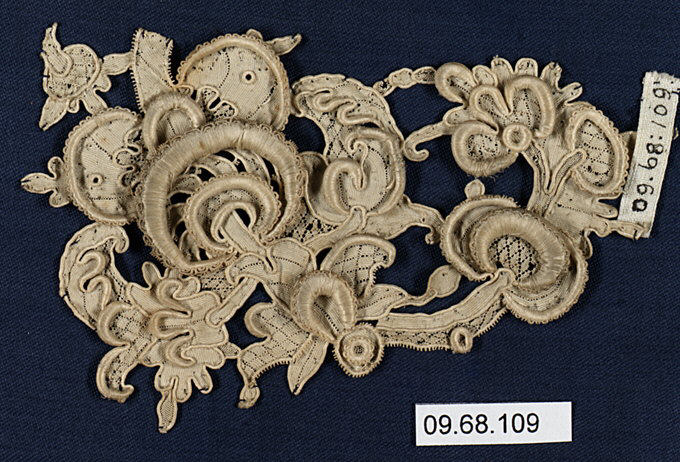The photograph depicts a carefully staged, full-color image of an ornate, abstract scroll design crafted from light gold or cream cloth set against a dark blue fabric background. This intricate piece, resembling an antique applique, is adorned with intricate lace and threaded details, forming interconnected horseshoe-like shapes that make it appear both whimsical and elegant. The fabric background and ornate design suggest it might have been part of a dress, uniform, or furniture adornment, possibly from the 1800s. Two visible tags provide an identifier: a worn, printed one in the top right corner reading "09.68.109" and a newer, embroidered tag sewn directly onto the piece with the same catalog number. This identifier suggests the item is part of a museum or inventory collection. The photograph, taken indoors under artificial light, captures the delicate, faded beauty of the cloth, highlighting its historical and decorative significance.